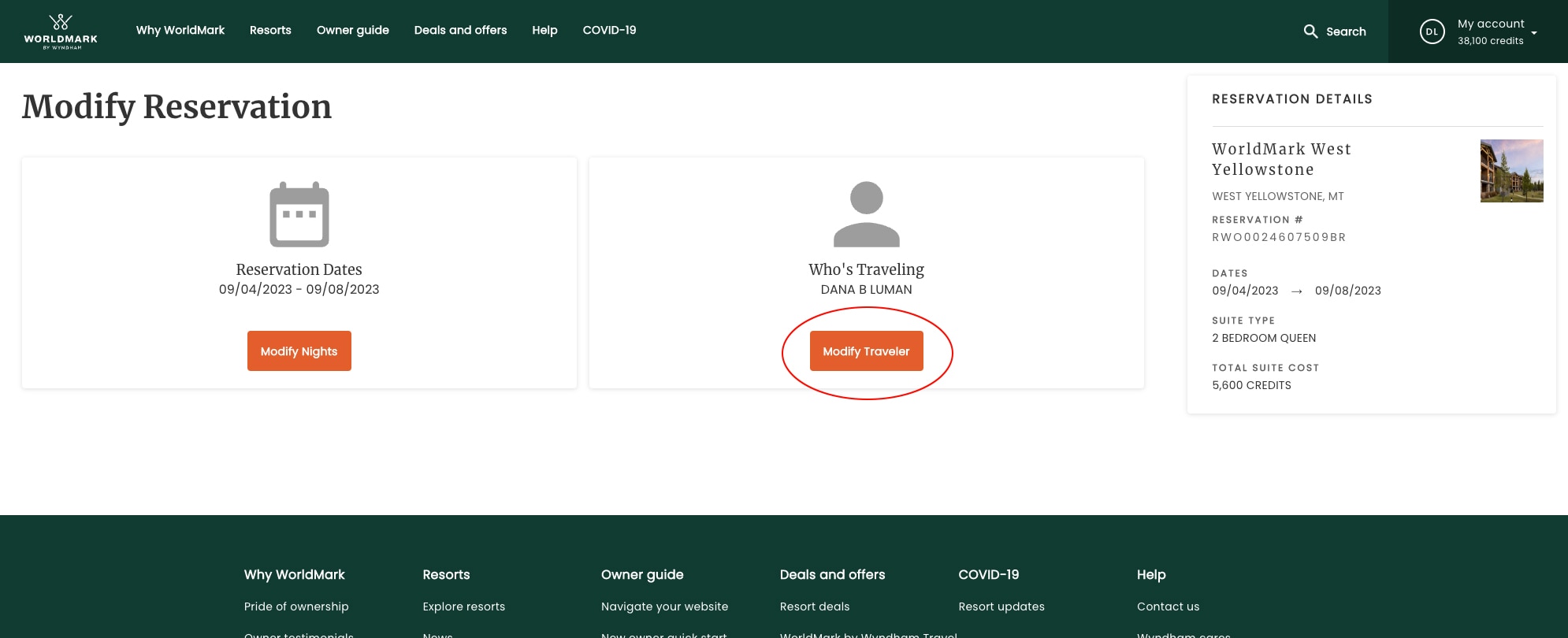This web page for a reservation from Worldmark features a logo in the top-left corner, which reads "Worldmark" against a dark green banner. To the right of the logo, there are several navigation links including "Why Worldmark," "Resorts," "Owner Guide," "Details and Offers," "Help," and "COVID-19." On the far right of the green banner, there's a search button, and further to the right, a "My Account" dropdown menu for users to sign in.

Centered on a white background in the middle of the page is the section titled "Modify Reservation." Directly beneath this title, it states the reservation dates as "9-4-2023 to 9-8-2023," accompanied by an orange "Modify Nights" button. To the right, there's a section labeled "Who's Traveling?" listing the name "Dana B. Laman," with an adjacent orange "Modify Traveler" button that is circled in red, indicating it's highlighted for emphasis.

To the right of the "Who's Traveling?" section is the "Reservation Details" for "Worldmark West Yellowstone," accompanied by a picture of the hotel's exterior. The bottom of the page features another dark green banner containing various informational links related to the website and the business.